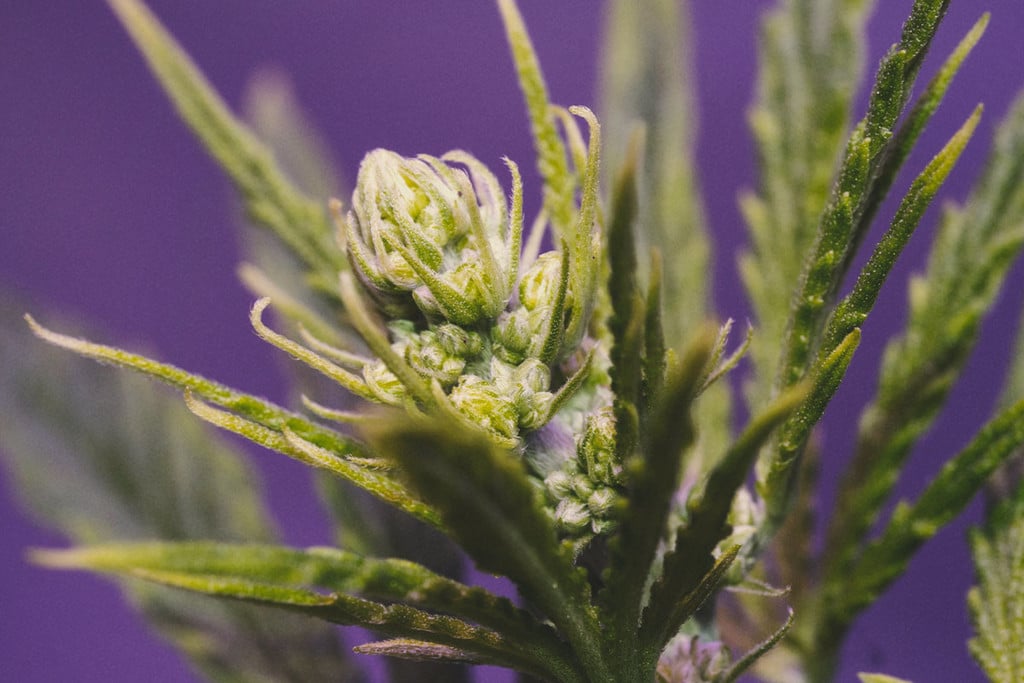This image is a very close-up photograph of a marijuana plant bud against a solid, out-of-focus purple background. The plant features an intricate cluster of light green buds adorned with thin, spiky leaves that have jagged, almost serrated edges. The buds display a combination of lime green, dark green, white, and occasional hints of purple, particularly at the tips. Small white hairs can be seen protruding from the buds, suggesting they are not yet in full bloom. Some leaves and parts of the plant in the foreground and background are out of focus, drawing attention to the vivid and detailed central bud, giving the image depth and texture.